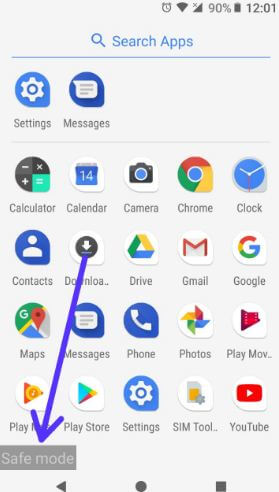This image displays a screenshot of a cell phone's user interface, specifically showcasing the app drawer with a search functionality. The top portion of the screen features the typical status bar icons, indicating the device is connected to Wi-Fi and mobile network with full signal strength, and showing the current time and battery level.

Beneath the status bar lies a prominent search bar labeled "Search apps," designed to facilitate easy navigation through the numerous applications installed on the device. The main display area is organized with app icons arranged in a grid format, spanning several rows.

The first visible row contains icons for essential system applications: Settings and Messages. Proceeding to the next row, left to right, we observe icons for the Calculator, Calendar, Camera, Chrome browser, and Clock applications.

The subsequent row includes Contacts, Downloads, Drive (Google Drive), Gmail, and Google apps. Following this row, the icons for Maps, Messages (again), Phone, Photos, Play Movies, Play Music, Play Store, Settings, SIM Tools, and YouTube are displayed, indicating a comprehensive collection of both utility and entertainment applications.

A notable feature at the bottom of the screen is a gray box labeled "Safe mode," with a downward-pointing arrow highlighting it. Safe mode is a diagnostic mode typically used to troubleshoot issues by loading only essential system applications.

Overall, the image offers a detailed view of a cell phone's app drawer in safe mode, complete with a well-organized layout of commonly used applications.